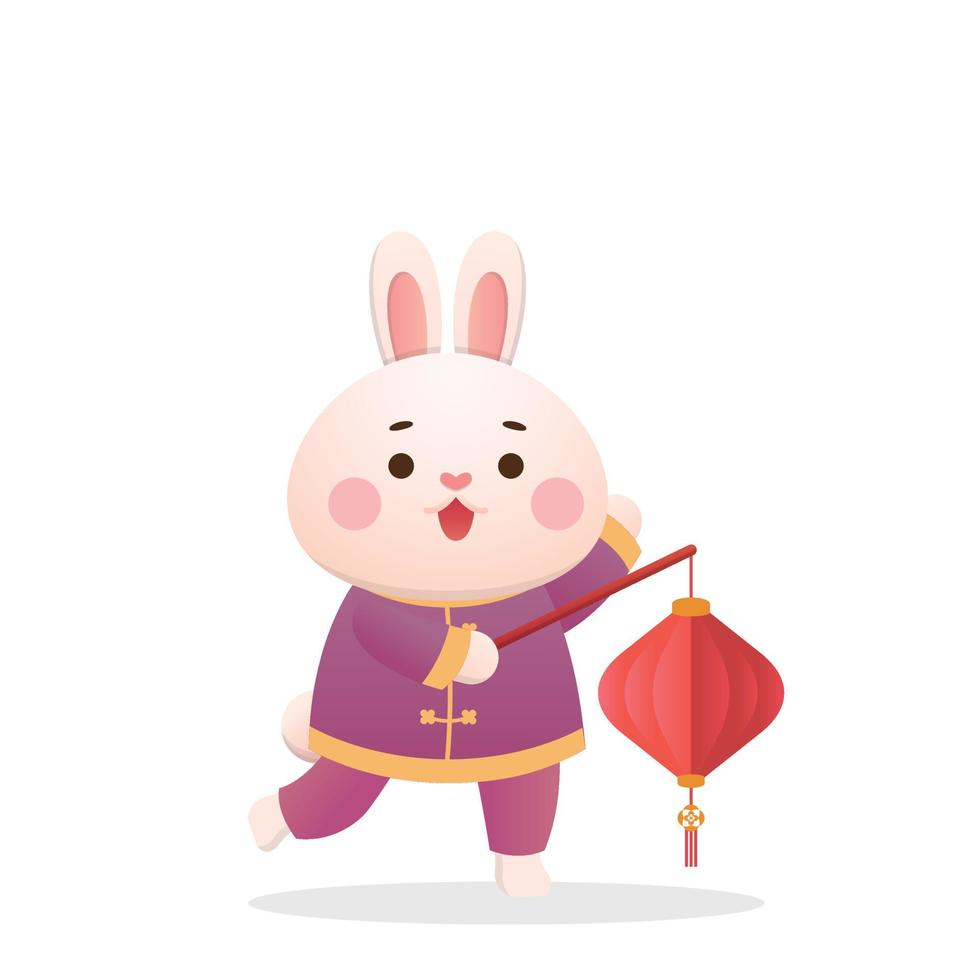This detailed digital illustration features a lively pink rabbit, standing upright on its two hind legs in humanoid fashion. The rabbit has prominent, round brown eyes with playful brown eyebrows, a small heart-shaped pink nose, and a darker pink tongue peeking out from its open mouth, which adds to its cheerful expression. Its ears are pointed straight up from the top of its head, and they, along with its cheeks, are colored a deeper pink, giving the rabbit a blushing, animated appearance.

Donning traditional Chinese attire, the rabbit is dressed in a vibrant purple jacket with ornate gold trim and decorative gold buttons. The bottom of the jacket and the wrists of the sleeves are also adorned with a gold lining, which provides a regal touch. From underneath the sleeves, the rabbit's white paws emerge. Complementing the jacket, the rabbit sports matching purple pants, through which its feet and small tail are visible.

In its right hand, the rabbit holds a red lantern with intricate gold accents, which dangles from a brown stick. This lantern is attached by a red rope and features small decorative elements hanging from the bottom. The rabbit's left hand is raised, contributing to the dynamic feel of the illustration, and its right leg is lifted backward, as if in mid-motion. A subtle gray shadow beneath the rabbit adds depth to the image, enhancing the sense of action and liveliness in this anthropomorphic character.